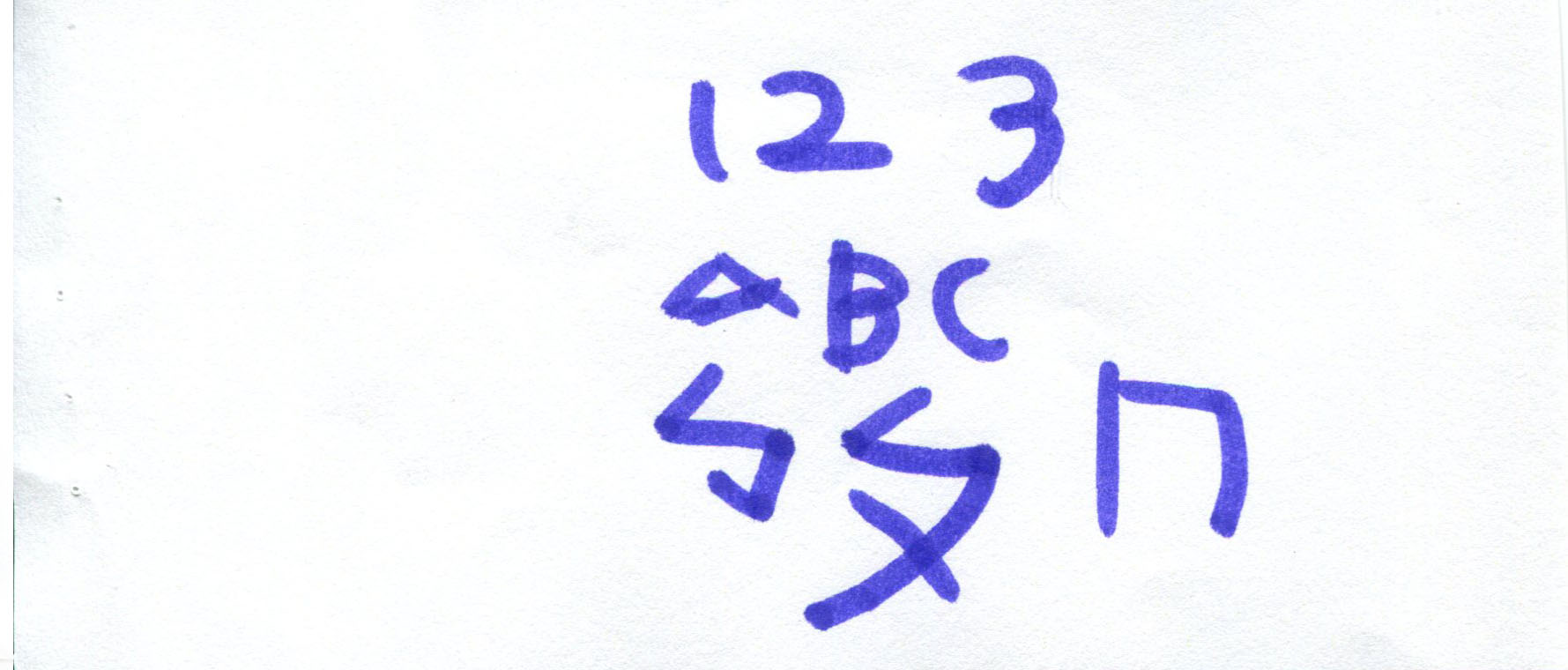This photograph features a white piece of paper covered with characters drawn in blue marker. The arrangement consists of three rows, each containing three characters. 

In the first row, we see numeric digits: "1," "2," and "3" sequentially. The second row comprises uppercase alphabetic letters: "A," "B," and "C." 

The third row is more intriguing, showcasing a series of symbols rather than standard alphanumeric characters. The first symbol resembles a lightning bolt with a zigzag pattern similar to the letter "Z," but it includes an additional upward line. The second symbol appears to be a variation of the first but morphs into a shape that intersects to form an "X" or an elongated "V" at its base, giving it a more complex form. The final symbol in the row might be interpreted as a squared-off, lowercase "n," but its geometric precision suggests it might be a different symbol altogether, characterized by its atypical, angular structure. 

This interplay of numbers, letters, and ambiguous symbols creates a visually engaging and thought-provoking composition.